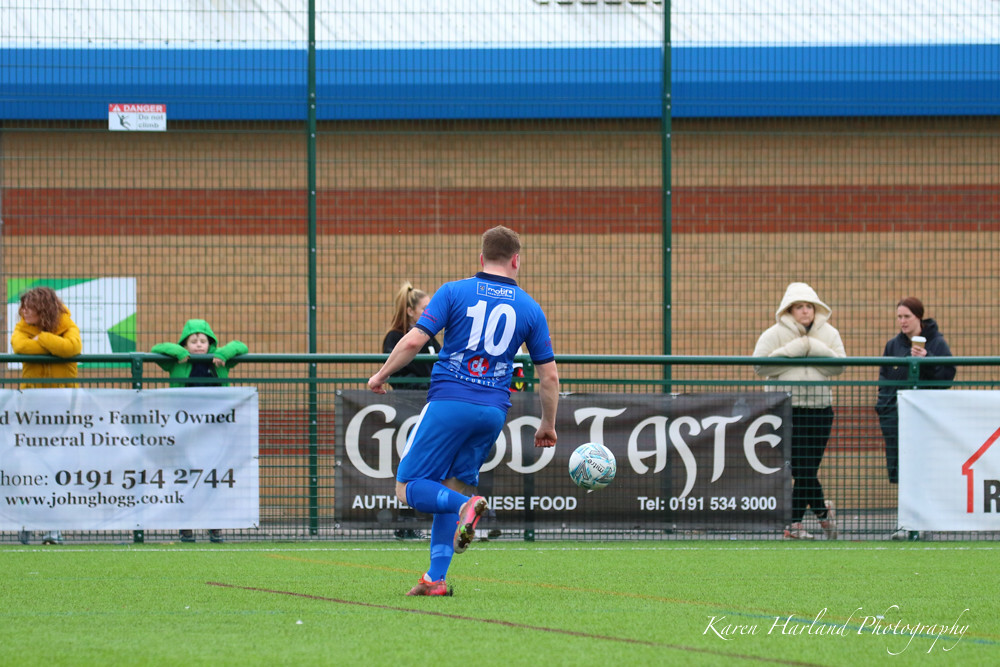In a daytime outdoor soccer game depicted in a landscape photograph by Karen Harland Photography, we see a male player, wearing a blue jersey with the number 10, blue shorts, and matching blue shin guards. His cleats are reddish on the bottom and brown on top, creating a bright contrast to his uniform. The player, who has very short light brown hair, is in mid-action: his right leg is firmly planted on the green field while his left leg is raised behind him at a right angle, suggesting a dynamic movement to the right. His body is slightly leaned to the right, with his right arm lower and his left arm slightly raised, indicating he is preparing to turn. In the bottom right-hand corner, the photograph is marked with "Karen Harland Photography" in white print, indicating it has been edited or professionally taken. In the background, a chain-link fence stands with several banners draped across it. The left banner reads "Winning Family Owned Funeral Directors" with a UK-based website, implying the scene is set in the United Kingdom. The middle banner advertises "Good Taste Authentic Chinese Food," and a partially visible right banner features a house symbol. Behind the fence, a building is visible, adding depth to the setting. The overall image captures the intensity and focus of the player amidst a backdrop of local advertisements and spectators.